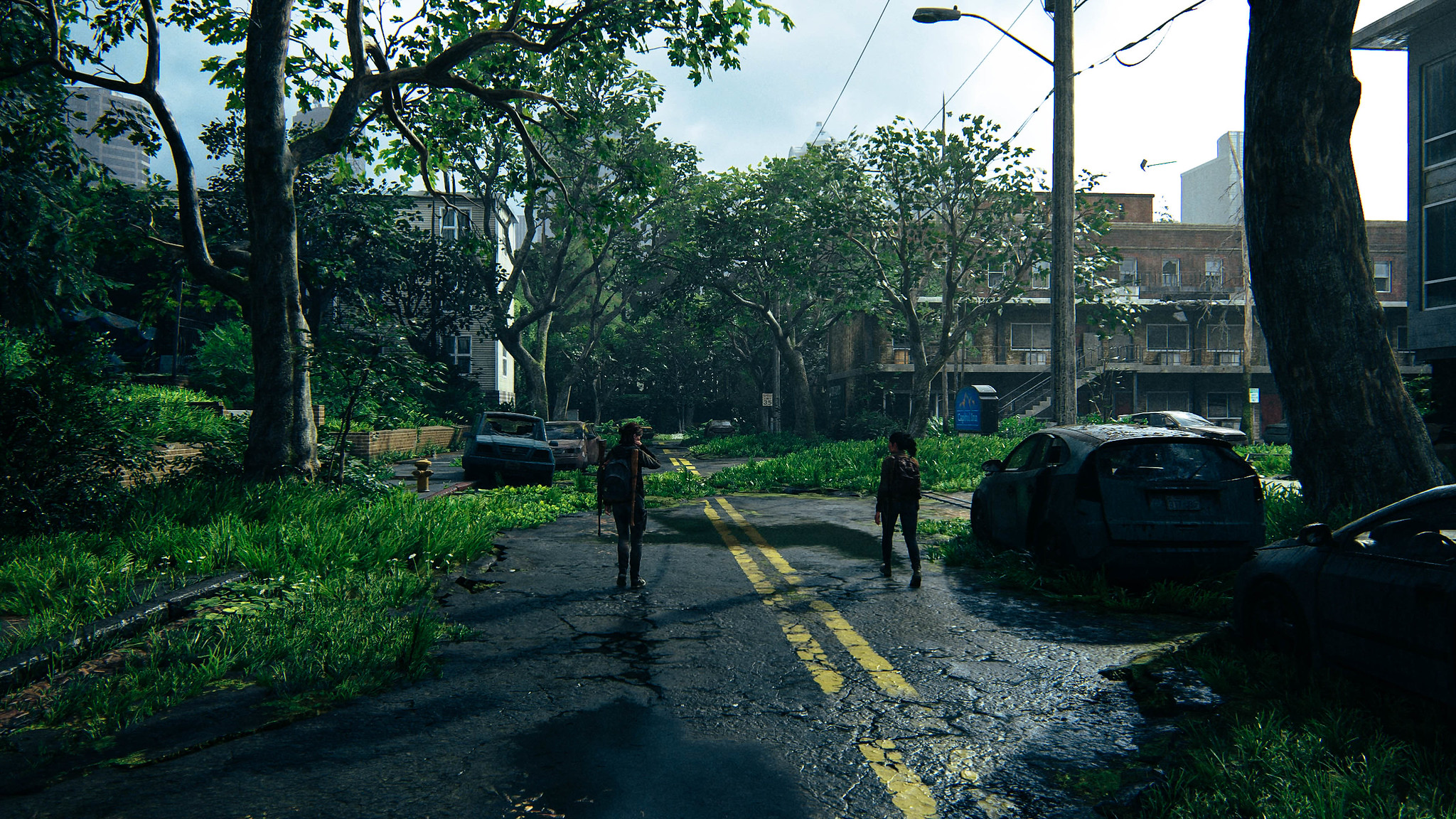This image is a screenshot from a highly detailed, almost photorealistic 3D game set in a post-apocalyptic or abandoned neighborhood. Dominating the foreground is an old asphalt street marked by two yellow lines running down the center, extending into the distance. The road appears aged and unkempt, with grass breaking through the asphalt and taking over the edges.

Two figures, a young male on the left and a young female on the right, stand on the road. They are almost silhouetted due to the harsh shadows that dominate the scene. To the right of the road, abandoned cars are parked, overtaken by invasive grass and appearing dirty.

A variety of structures populate the scene: a tree and several buildings, including an apartment complex in the background on the right. The right side of the road is lined with light posts and electrical poles, their power lines trailing along the street.

The left side of the image features a dense growth of vibrant, uncut green grass and more trees, partially obscuring houses further back. Additional abandoned cars are visible further down the road, adding to the desolate atmosphere. The sky is partly cloudy, indicating daytime, casting a natural light over this eerily deserted neighborhood.